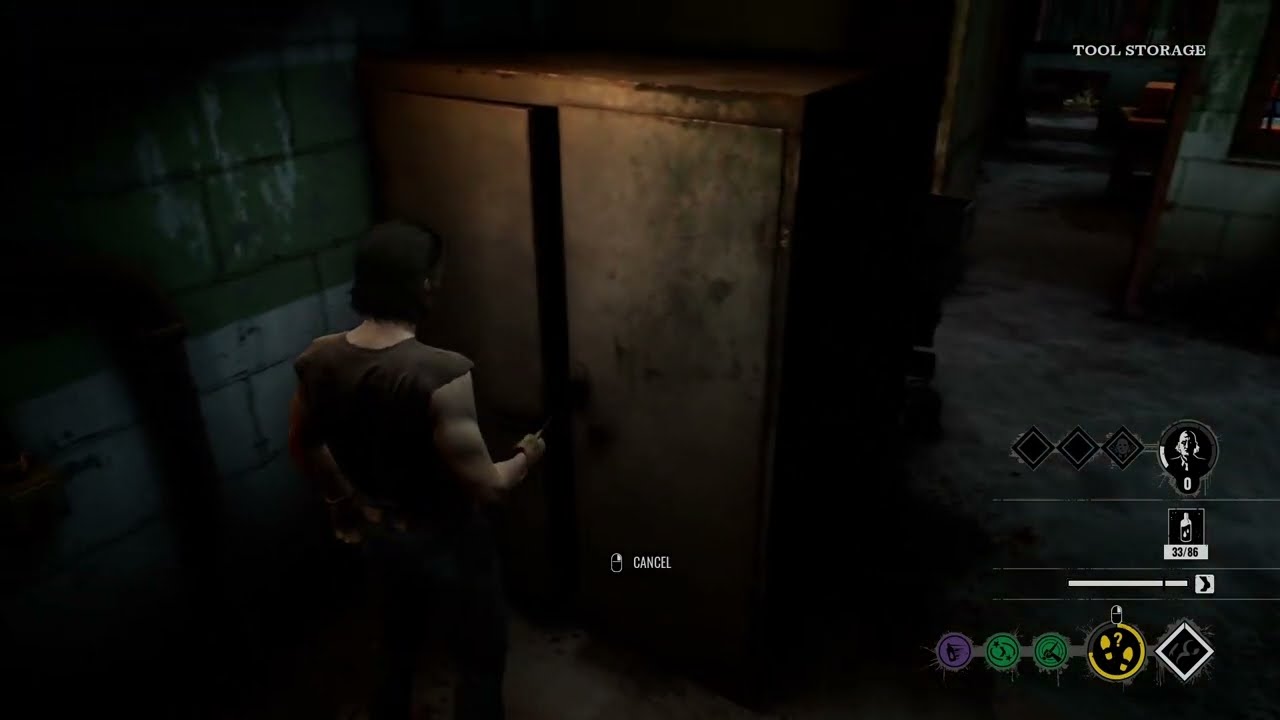This image appears to be a still from a third-person video game, reminiscent of titles like "Splinter Cell." The setting is a dimly lit, dirty, and worn-down basement. The walls are made of large bricks, with the lower half painted white and the upper half painted green, where the paint is peeling. The floor is dark gray concrete, and dim overhead lighting casts a bleak atmosphere.

In the scene, a white male character with black hair that is almost shoulder-length stands slightly left of center, facing a rusted metal or stained wooden cabinet with its door partially open. He wears a dark, sleeveless shirt, making him look ready to engage with his environment. To his right, a long, shadowy hallway stretches out, supported by stone columns.

Text elements enhance the game interface: "Tool Storage" appears in the top right corner, and in the bottom right corner, there are various icons for menu options and item selections. Just below the center of the screen, a cursor is accompanied by the action label "Cancel," indicating an available game action.